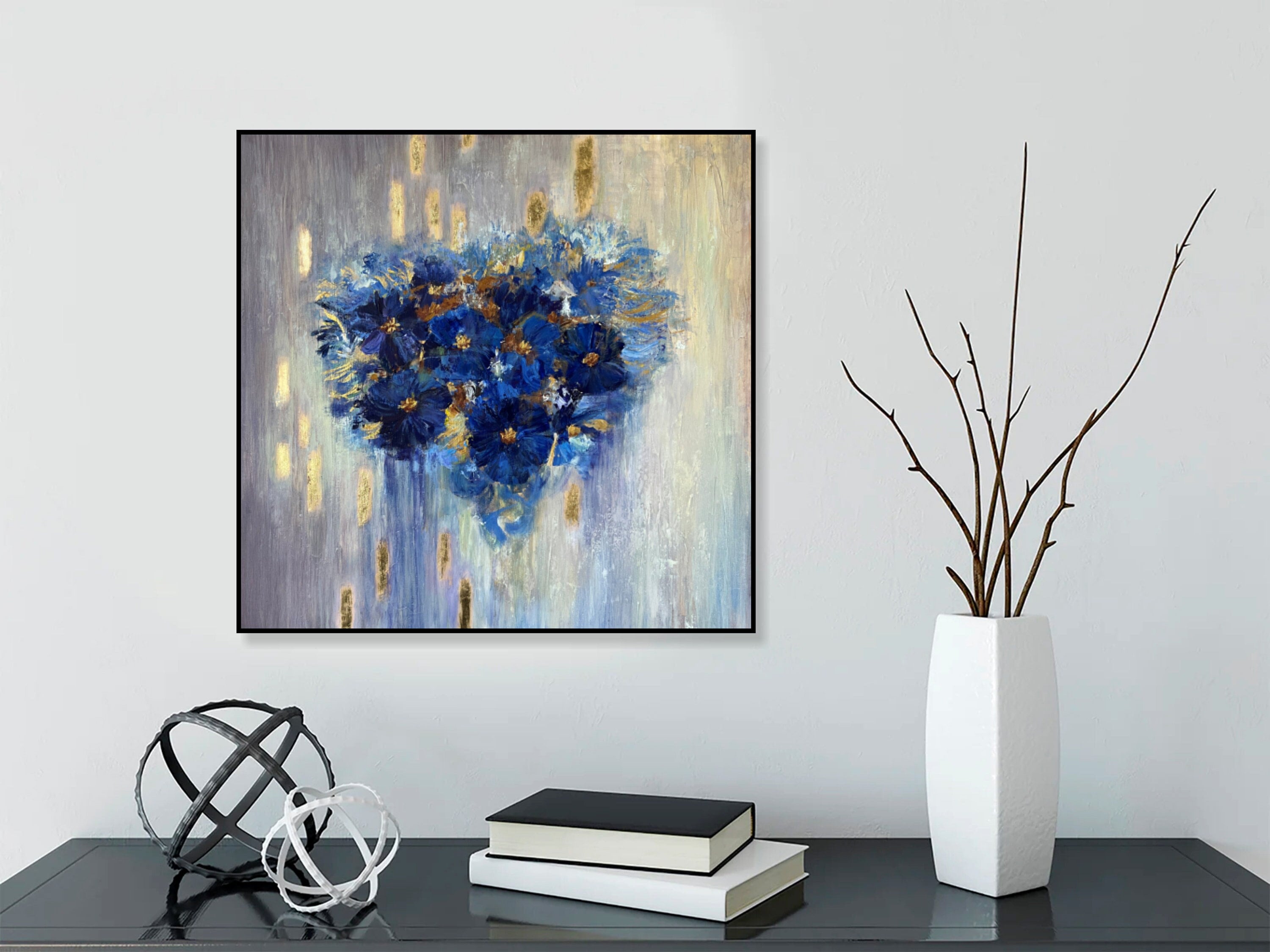The image showcases a beautifully detailed painting of blue flowers with delicate gold accents, nearly forming the shape of a heart, with light blue flowers gracing the edges. The backdrop is an intricate blend of gray, white, yellow, and blue with cascading gold specks that add a touch of elegance. The painting is elegantly presented on a white wall, and placed below it is a sleek black table that enhances the minimalist aesthetic. The table features an array of monochrome decor: a white vase with bare branches, two metallic spheres—one larger black sphere and a smaller white one resembling an atom symbol—along with a pair of books, one black and one white, arranged inversely to the spheres. The overall setting emphasizes the painting, making it the focal point of the composition, while the sophisticated decor complements its artistic appeal.